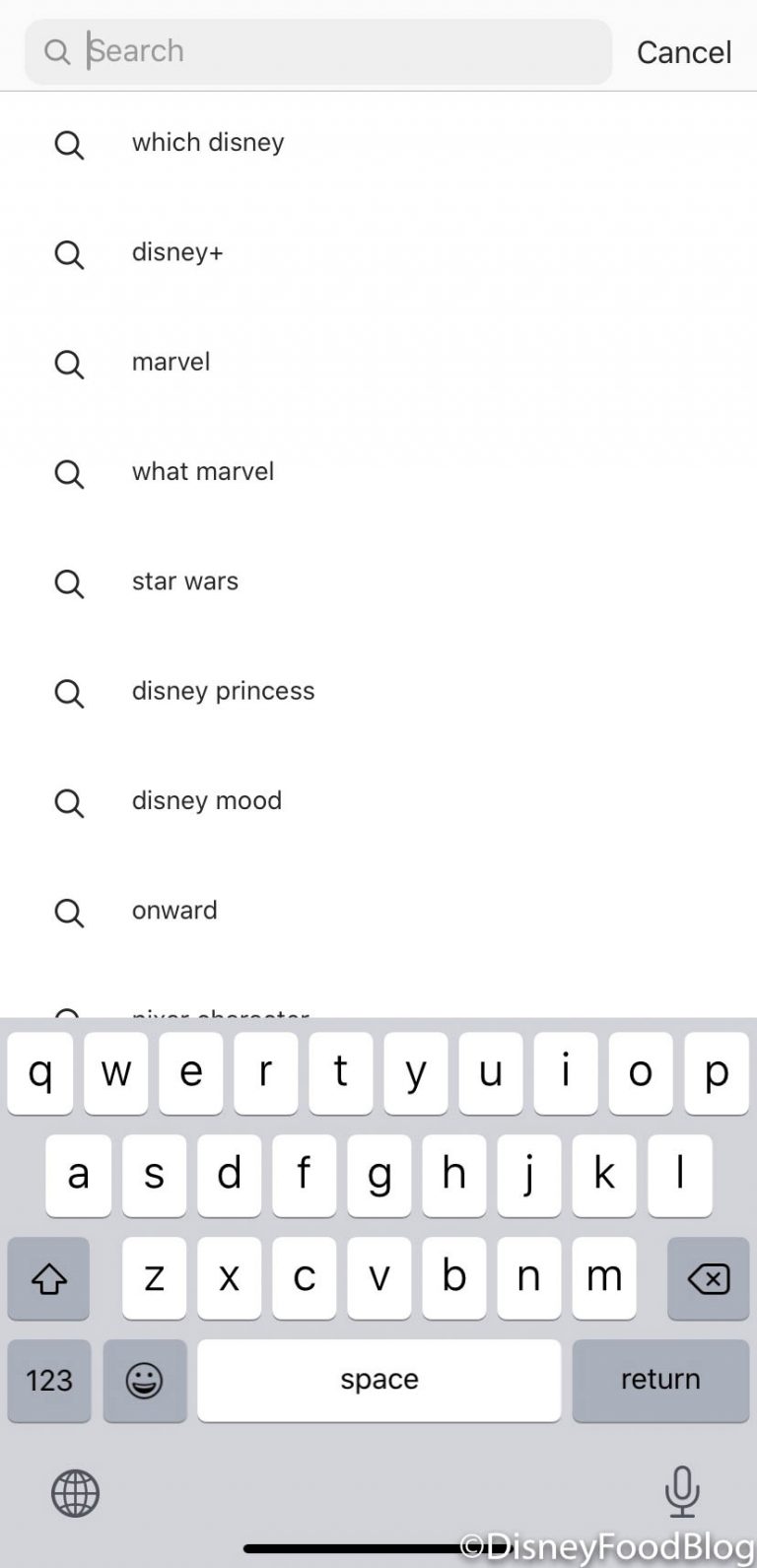This screenshot captures the search interface of a mobile application. At the top of the screen, there's a search bar featuring a small magnifying glass icon, followed by a "Cancel" button. The search bar contains the placeholder text "Search," indicating that the user has clicked into it, causing several suggestions to appear below. These suggestions include categories like Disney, Disney Plus, Marvel, Star Wars, Disney Princess, Disney Mood, Onward, and Disney Food Blog.

Below these search suggestions is an on-screen keyboard, which is displayed for user input. The keyboard features black letters on white keys, set against a grey background. Each word in the search suggestions has a small magnifying glass icon next to it, indicating it as a searchable term.

The keyboard itself includes various functional keys such as an upward-pointing arrow for capitalization, a "123" key for switching to numeric input, a smiley face key for emoticons, a "Return" key, and a delete key. The bottom part of the screen fades to a lighter grey, providing a subtle contrast to the rest of the interface.